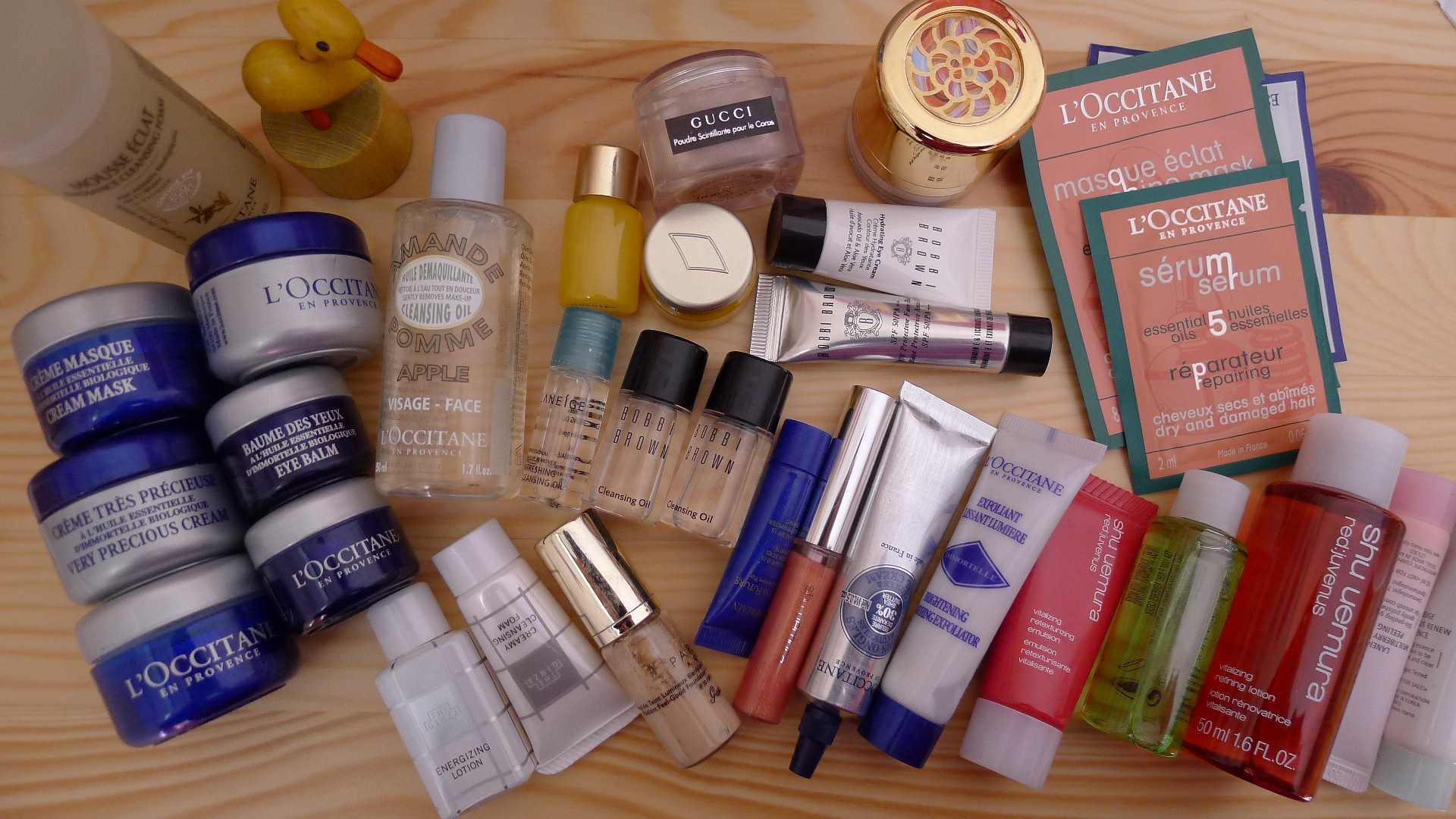This detailed photograph features an array of beauty products carefully arranged on a rustic wooden surface, predominantly comprised of sample-sized items. 

**Top Left Section:**  
- **White Bottle:** A white bottle labeled "E-Clack" (label is unclear)
- **Wooden Ducky:** A charming wooden duck on a stand adds a whimsical touch.

**Middle Left Section:**  
- **L'Occitane Products:** Six small jars from L'Occitane, housing various eye balms, face creams, and masks. These jars sport a mix of blue and silver lids along with corresponding colored bodies, creating a visually appealing assortment.

**Center Section:**  
- **Cleansing Oil:** A distinctive bottle of apple-scented cleansing oil from L'Occitane.
- **Three Small Bottles:** Clear bottles with unspecified contents.
- **Various Tubes:** 
  - A white tube
  - A small white bottle
  - Another tube with a gold cap

**Right Section:**  
- **Blue Tube:** A generic blue tube.
- **Pink Lip Liner:** A lip liner that stands out with its pink hue.
- **Additional L'Occitane Products:** More items featuring blue lids and bodies.
- **Shu Uemura Items:** 
  - A pink product labeled Shu Uemura
  - A yellow-colored substance in a small bottle
  - Another Shu Uemura product, likely a cleanser.

**Top Right Section:**  
- **Paper Samples:** Pink serum sample packets by L'Occitane.
- **Gold Container:** Possibly a powder product.

This collection meticulously showcases a variety of skincare essentials, predominantly highlighting the luxurious offerings from L'Occitane, interspersed with items from other renowned brands like Shu Uemura.